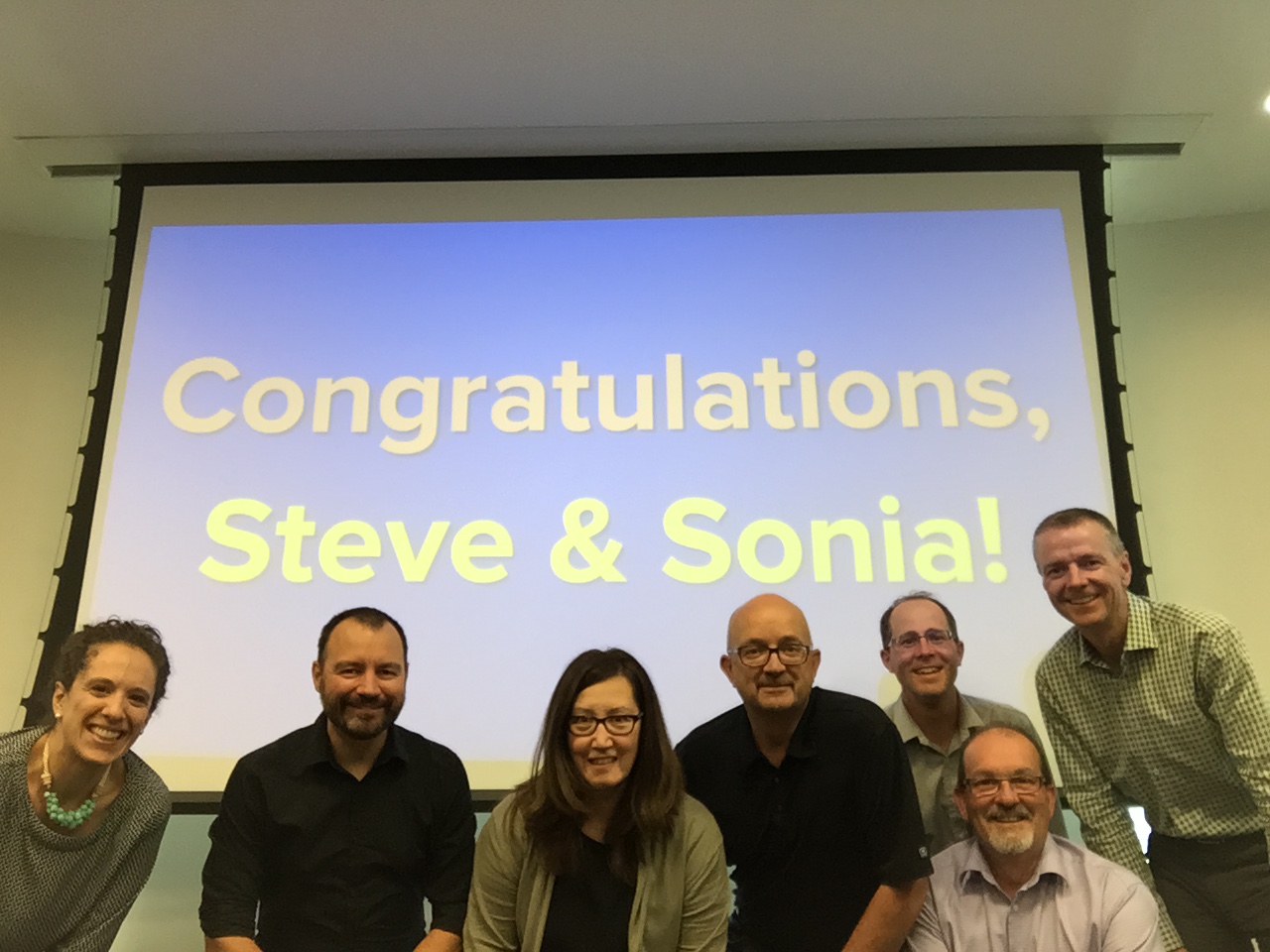In an indoor setting that appears to be a meeting or conference room, seven individuals are posed in front of a large projector screen. The screen displays a celebratory message with a blue background and orange-yellow text, reading, "Congratulations, Steve and Sonia." The group consists of two women and five men, all seemingly in their late 50s to early 60s, suggesting a more mature age group.

From left to right: the first woman is smiling and wearing a grey sweater paired with a beaded turquoise necklace. Next to her stands a man in a black button-down shirt. In the center stands another woman, also smiling, adorned in a green cardigan over a black shirt and wearing glasses. Adjacent to her is a balding man in a black golf shirt. Following him is a man in a dress shirt with a collar, accompanied by another man in a grey dress shirt with glasses and a white goatee. Finally, on the far right, a man is dressed in a checkered white and green dress shirt and slacks.

The setting, a room with a white ceiling and a partially visible pot light on the right side, along with a white wall, suggests this photograph captures a significant celebratory occasion, perhaps a retirement or a special recognition for Steve and Sonia.